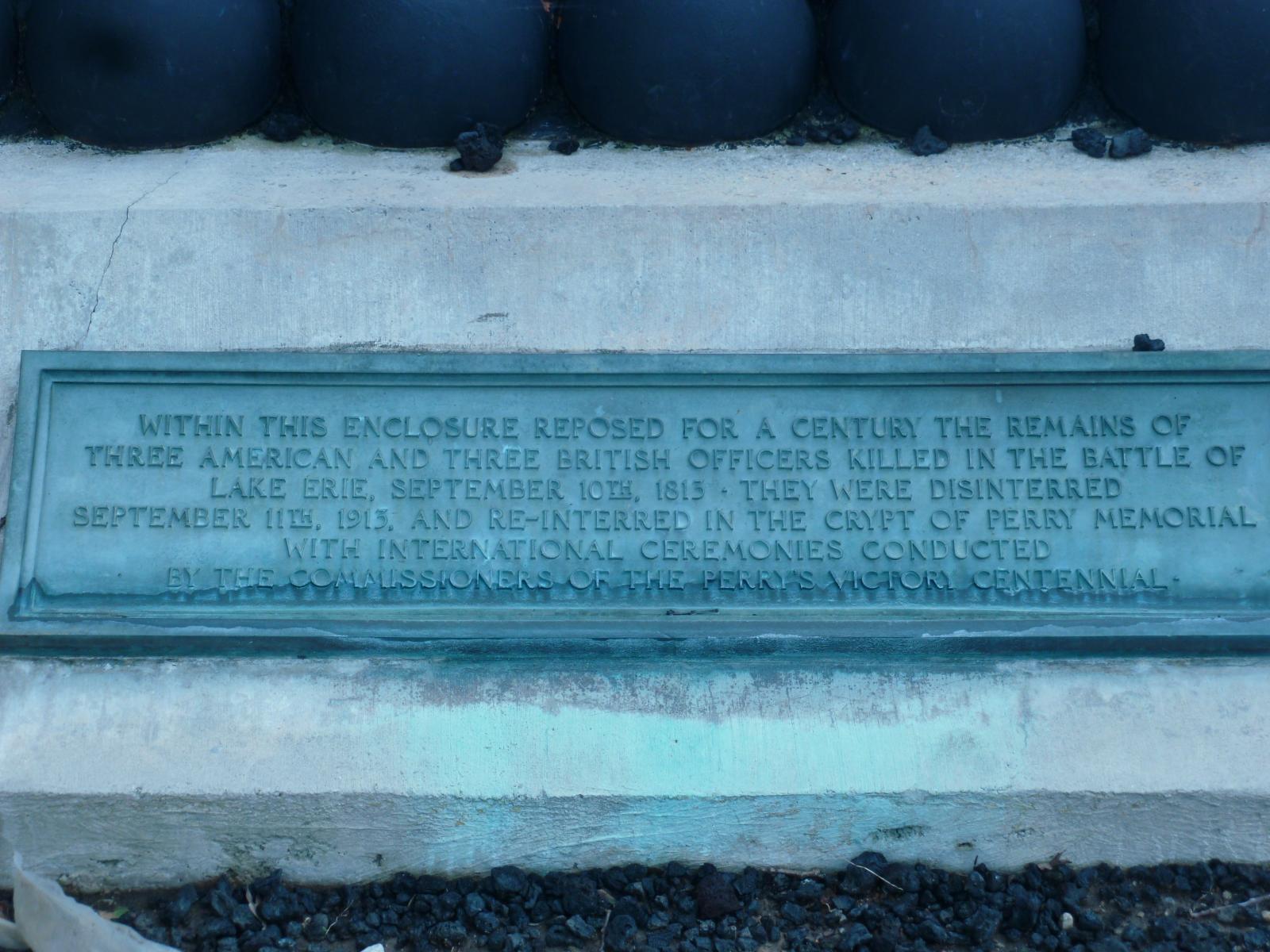This photo depicts a detailed stone monument, serving as a burial site memorial. The monument, constructed from concrete, features a prominent plaque made of metal with a greenish hue. This plaque is framed by gray and blue elements; the blue rectangle in the middle bears the inscription: "Within this enclosure reposed for a century the remains of three American and three British officers killed in the Battle of Lake Erie, September 10, 1813. They were disinterred September 11, 1913, and reinterred in the crypt of Perry Memorial with international ceremonies conducted by the Commission of the Perry's Victory Centennial." Surrounding the base of the monument are scattered black and blue pebbles and stones, some of which are placed atop the white section beneath blue circles, adding a poignant touch to the site.